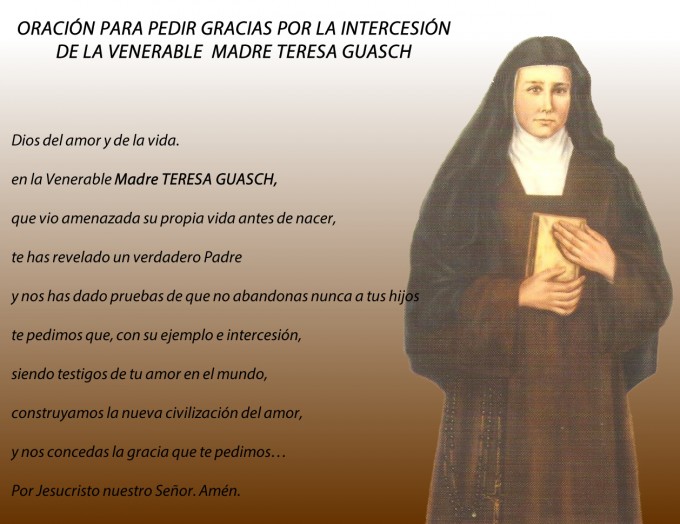The image depicts a religious-themed illustration with an ombre background that transitions from a light, almost white shade at the top to a darker brown at the bottom. In the upper left-hand corner, a title in Spanish reads "Oración para pedir gracias por la intercesión de la Venerable Madre Teresa Gouache." Along the entire left side of the image, a prayer written in Spanish features phrases like "Dios del Amor y de la Vida en la Venerable Madre Teresa Gouache." On the right-hand side, there is a detailed drawing of a solemn white nun wearing a black habit, a white high-collar shirt, and a long brown dress. She is looking straight ahead with a serious expression, clutching a book—presumably a Bible—against her chest, and a rosary is visible on one side of her dress. The image has the appearance of a slide that could be part of a presentation, like a Microsoft PowerPoint slide.